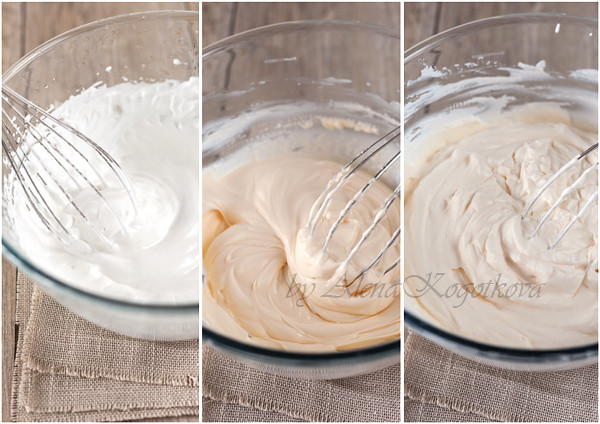A three-pane photograph presents different stages and angles of mixing within a clear glass bowl, captured against a tan dish towel background. Each panel showcases a distinct view of the bowl with a wire whisk involved in the mixing process. In the top panel, the whisk is positioned on the left side, and the mixture inside appears creamy, like egg whites or whipped cream. Moving to the middle panel, now viewed at a slightly different angle, the whisk is placed on the right-hand side, and the mixture seems more fluid and slightly orangish in hue. The bottom panel again shows the whisk on the right, depicting the mixture as thicker and lighter, signifying a progression in the mixing process. The sequence is unified by a tan dish towel background and a white watermark with gray text that reads, "by Elena Kagatskova," spanning across the center of the image.